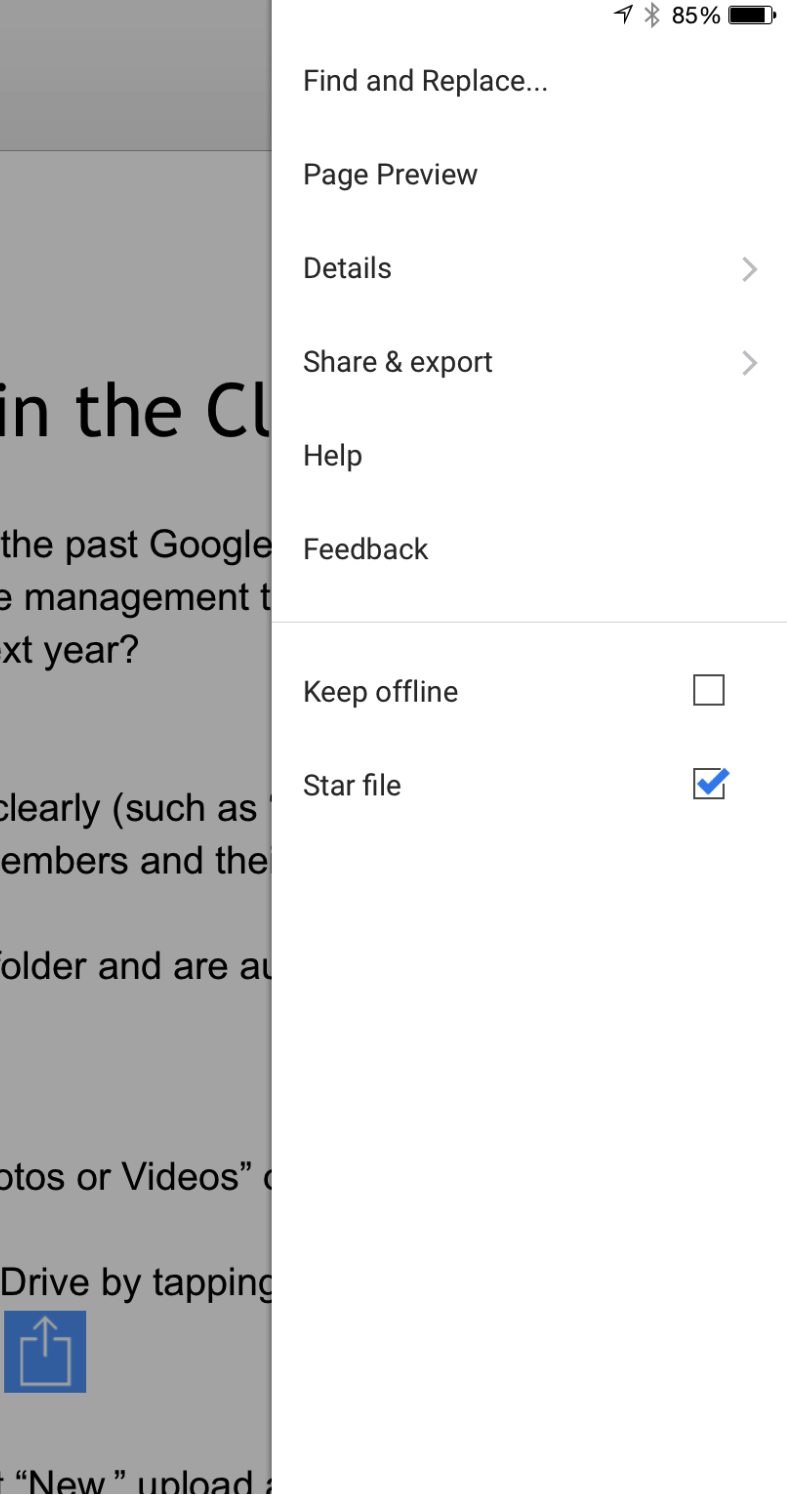The image captures a smartphone screen displaying an app interface. On the left side, a gray sidebar contains black text. Phrases such as "in the CU," and references to "past Google management," "members," "folder," "photos or videos," and actions like "drive by tapping new upload" can be seen. A blue "upload" button is partially visible.

The main screen shows a partially cut-off interface with the title bar at the top reading "Find and Replace..." along with options like "Page preview" and "Details," both with clickable arrows indicating further actions. Additional options such as "Share and export," "Help," "Feedback," "Keep offline," and "Star file" are listed. The "Keep offline" option is accompanied by an unchecked square, while the "Star file" option shows a blue-checked square, indicating it has been selected.